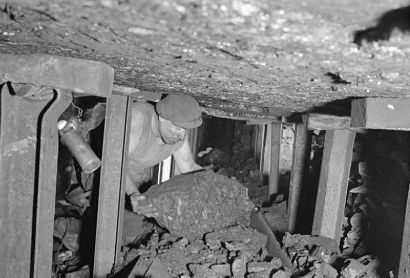This black and white photograph depicts a man working in what appears to be a confined, makeshift mine with a very low ceiling. The man, who has pale skin and a dirty face, is bent over due to the low height of the ceiling, and he is in the process of moving a large rock or possibly coal with his hands. He is dressed in a miner's outfit that includes a sleeveless shirt and a distinctive Jeff cap, reminiscent of styles common in the 1950s. The setting is supported by a combination of metal posts and wooden beams, providing structural support to prevent collapse. To the right-hand side of the image, there is a canister that may function as a light source. The ceiling above is soiled and cluttered with crumbled rocks, adding to the image's depiction of a laborious and rough environment. Overall, the photo exudes a sense of hard, grimy work common in early mining operations, with the worker seemingly engrossed in his gritty task.